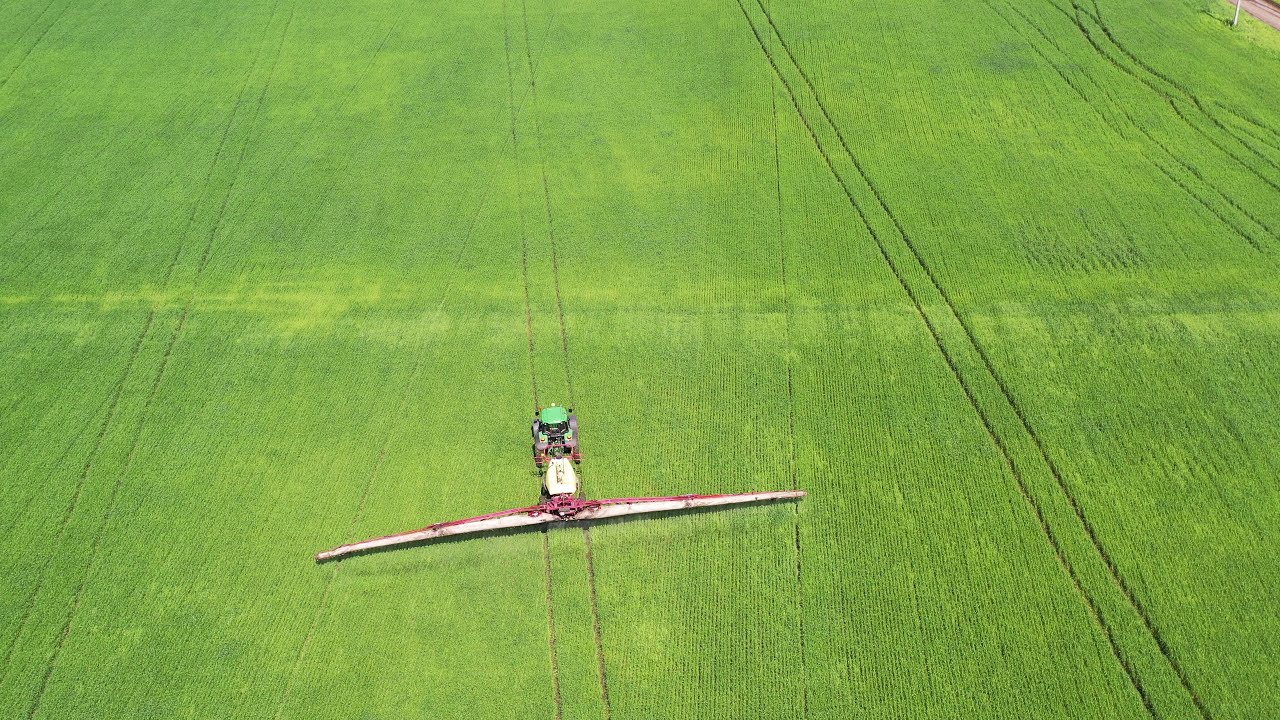In this aerial photo, we're looking down at a vast, lush green farm field that stretches out in all directions. Dominating the lower center of the image is a large tractor with a light blue upper section and elongated, horizontal arms that are red on top, white in the center, and black on the bottom, casting a shadow on the field. These arms extend widely to the left and right, creating a series of black parallel lines in the crops as the machine moves towards the viewer, indicating a systematic pattern of cultivation or treatment across the field. Numerous parallel lines are visible on both the far left and far right of the image, showcasing previous passes of the machine. To the top right corner, a small patch of brown suggests the presence of a road. It is unclear whether the tractor is mowing, gathering a crop, or perhaps spraying water or fertilizer. The overall view, potentially captured from a drone, plane, or helicopter, provides a comprehensive bird’s-eye perspective of the meticulous agricultural process taking place.